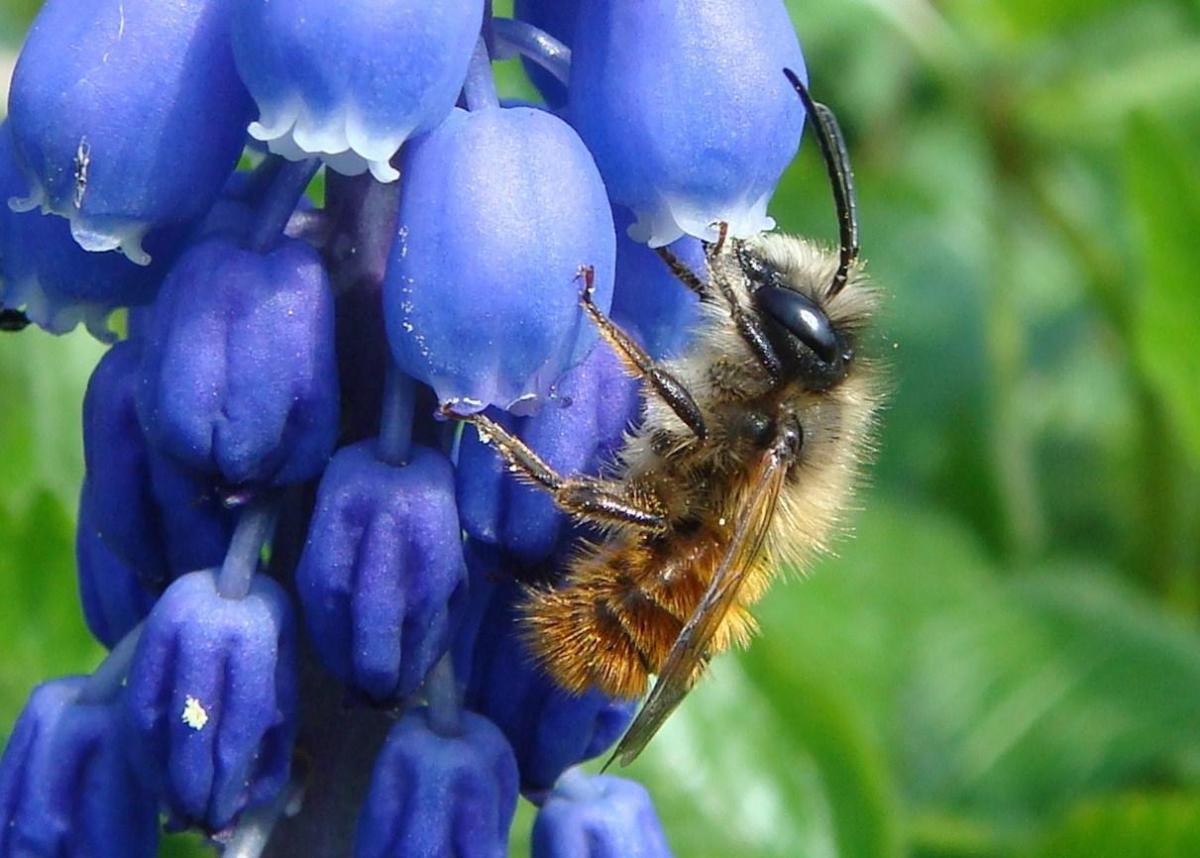In this detailed photograph, a fuzzy bee with a black head and tan, gold, and dark brown striped body is prominently featured. The close-up reveals the bee clinging vertically to two small, bell-shaped, blue-violet flower bulbs with white tips. Its six legs are firmly attached to the flowers, while its transparent wings, supported by visible spines, hang down. The bee's black antennae are visible as is one large eye reflecting sunlight. The flower bulbs, some of which are smooth and some crinkled, dangle like tiny peppers from blue stems. All of this is set against a blurred, grassy green background that provides a soft, bokeh effect.